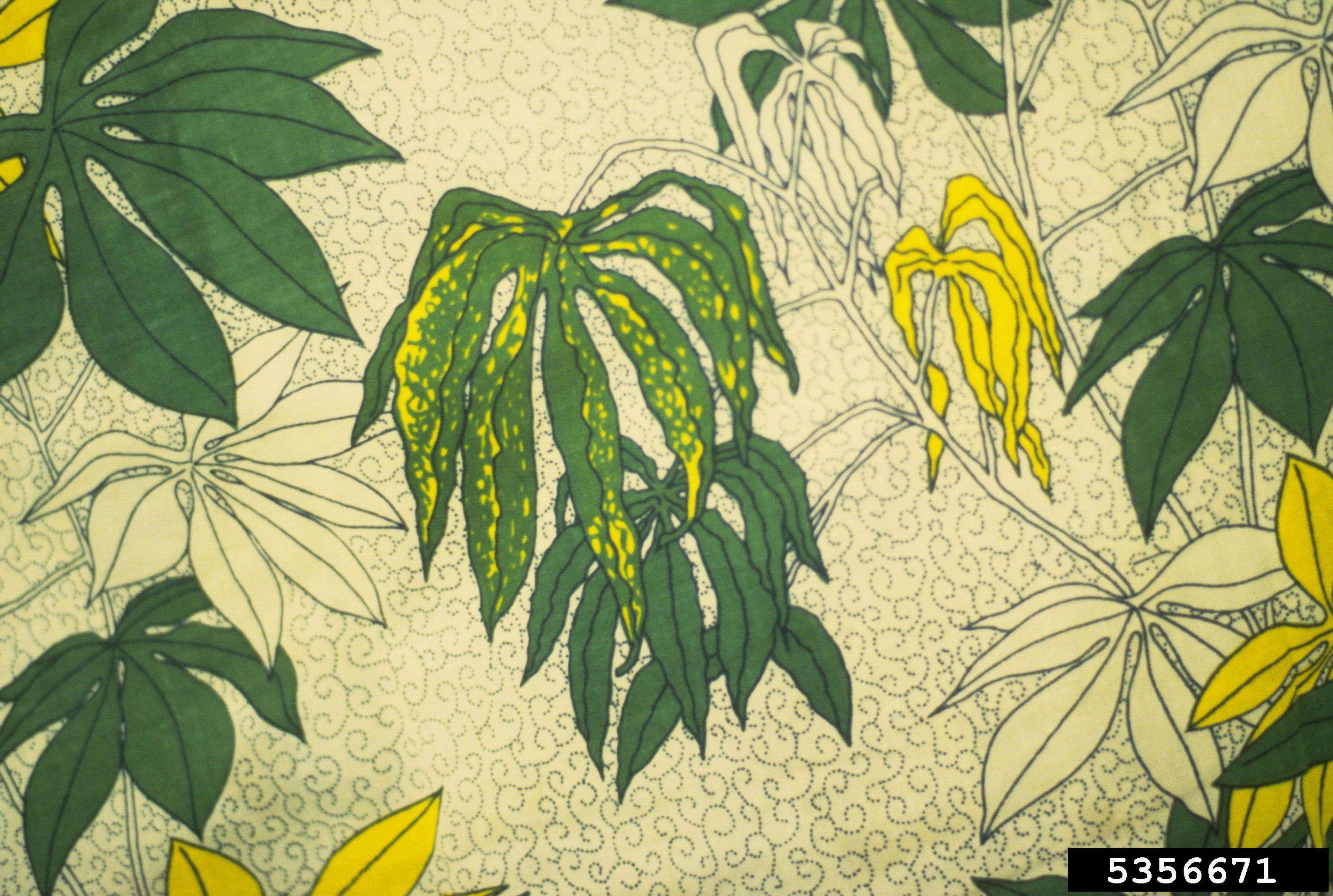This image depicts a detailed, artistic drawing that resembles a wallpaper swatch. The background is a cream color and features an assortment of leafy plants with varying fronds, each having six or seven extensions. The fronds vary in color from pale cream to green with yellow spotting, and some leaves are entirely yellow. The plant stems are left uncolored, creating a striking contrast. In the lower right corner, there is a small black rectangle with the white text "5356671" overlaid on the artwork. Behind the plants, a dotted, swirling, repeating gray pattern adds additional texture and depth to the image.